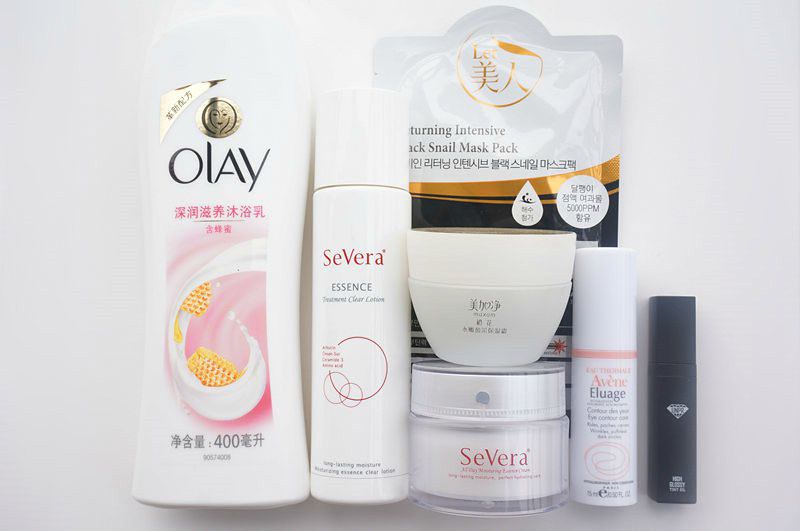The image showcases an array of beauty products in close-up detail, arranged neatly from left to right. On the far left, there is a container of Olay beauty cream, distinguished by its packaging featuring a cream swirl design set against a pink backdrop. The text on this packaging is in a language other than English. Next to it, the second product is packaged in white with striking red text that reads "Severa Essence." Adjacent to this, the third item is a glass jar also branded as Severa, with a white plastic jar placed on its lid. Continuing to the right, there is an elegantly designed foil package with white and black colors adorned with gold trim, labeled "Intensive Snail Mask Pack" in bold black text. Completing the arrangement, there are two additional tubes of beauty products, the details of which are not specified. The assortment provides a visually interesting display of varied beauty treatments and skincare solutions.